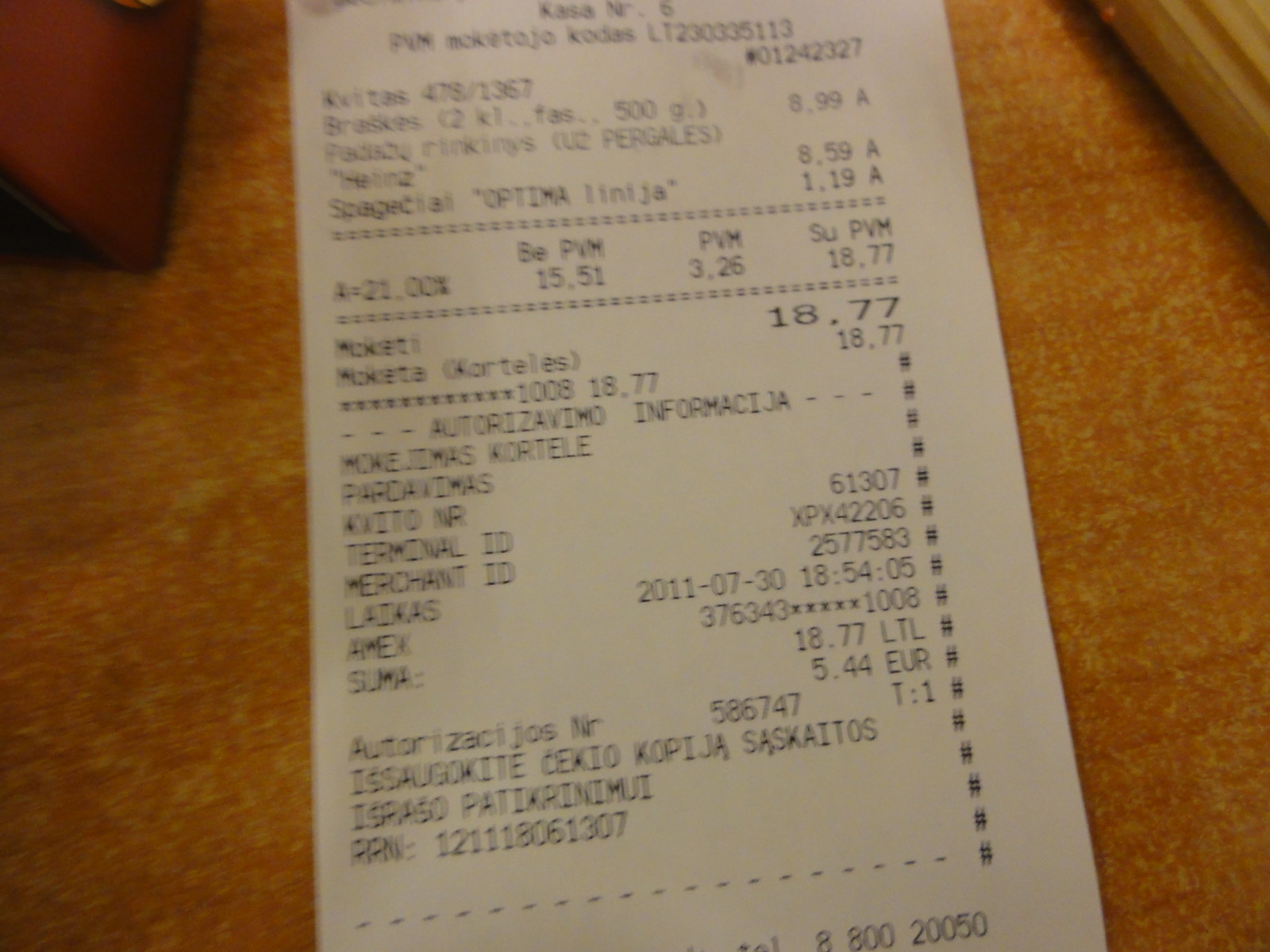The image is a close-up photograph of a register receipt placed on a light orangish wooden tabletop. The receipt is printed on white thermal paper with black text, written in a foreign, likely Slavic, language. The visible portions of the receipt include several numerical values: 899, 859, 119, 1551, 326, 1877, 61307, XPX42206, and the date 2011-07-30. The total amount listed on the receipt is 18.77, and it is additionally noted as 1877 LTL and €5.44, indicating a total of 18.77. The payment was made using an American Express card, with the authorization number 586747. The receipt has more detailed information than typical receipts in the United States.